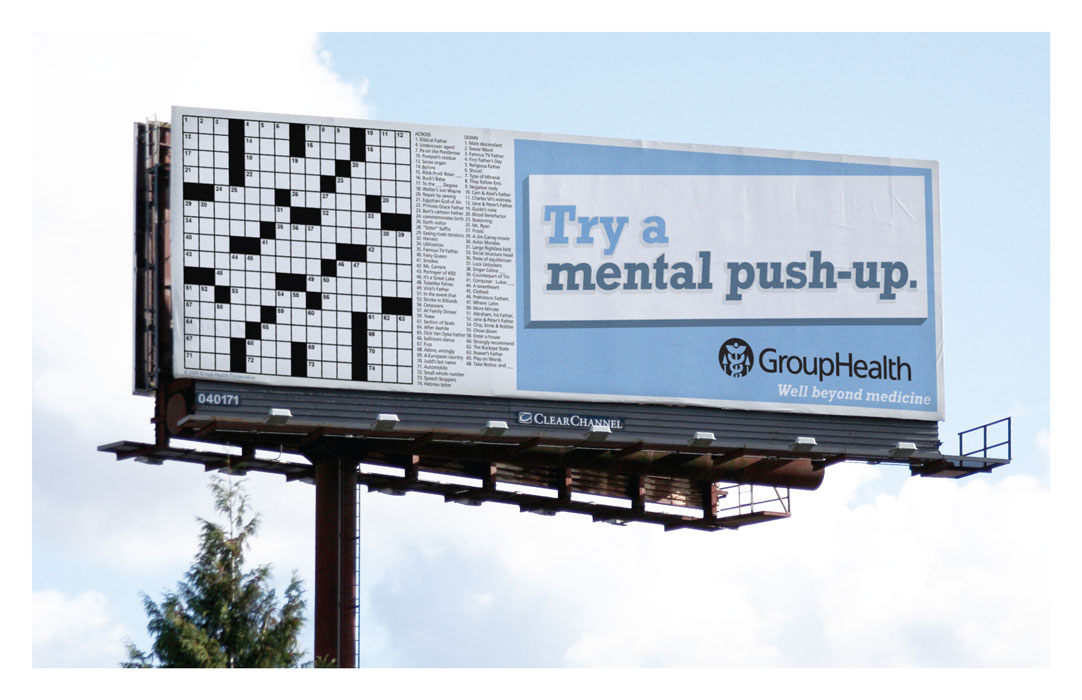The image depicts a large billboard set against a clear blue sky, with a significant cloud positioned in the upper left corner and another smaller cloud in the bottom right corner. On the bottom left, there's a tall green tree with its leafy top visible. The billboard, mounted on a thick brown pole, is much wider than it is tall and has a ladder attached to its support structure.

On the left half of the billboard, there is an empty black-and-white crossword puzzle grid with a number of small, unreadable clues listed to the right side of the grid. The right half of the billboard features a blue background with a white rectangular text box. Inside this text box, it reads "Try a mental push-up" in a combination of light and dark blue text. Below this, there's a medical symbol that resembles a staff with two snakes winding around it, followed by two arrows pointing to the right. The text "Group Health well beyond medicine" is written underneath this symbol. The backside of the billboard, facing the opposite direction, is not visible in the image.